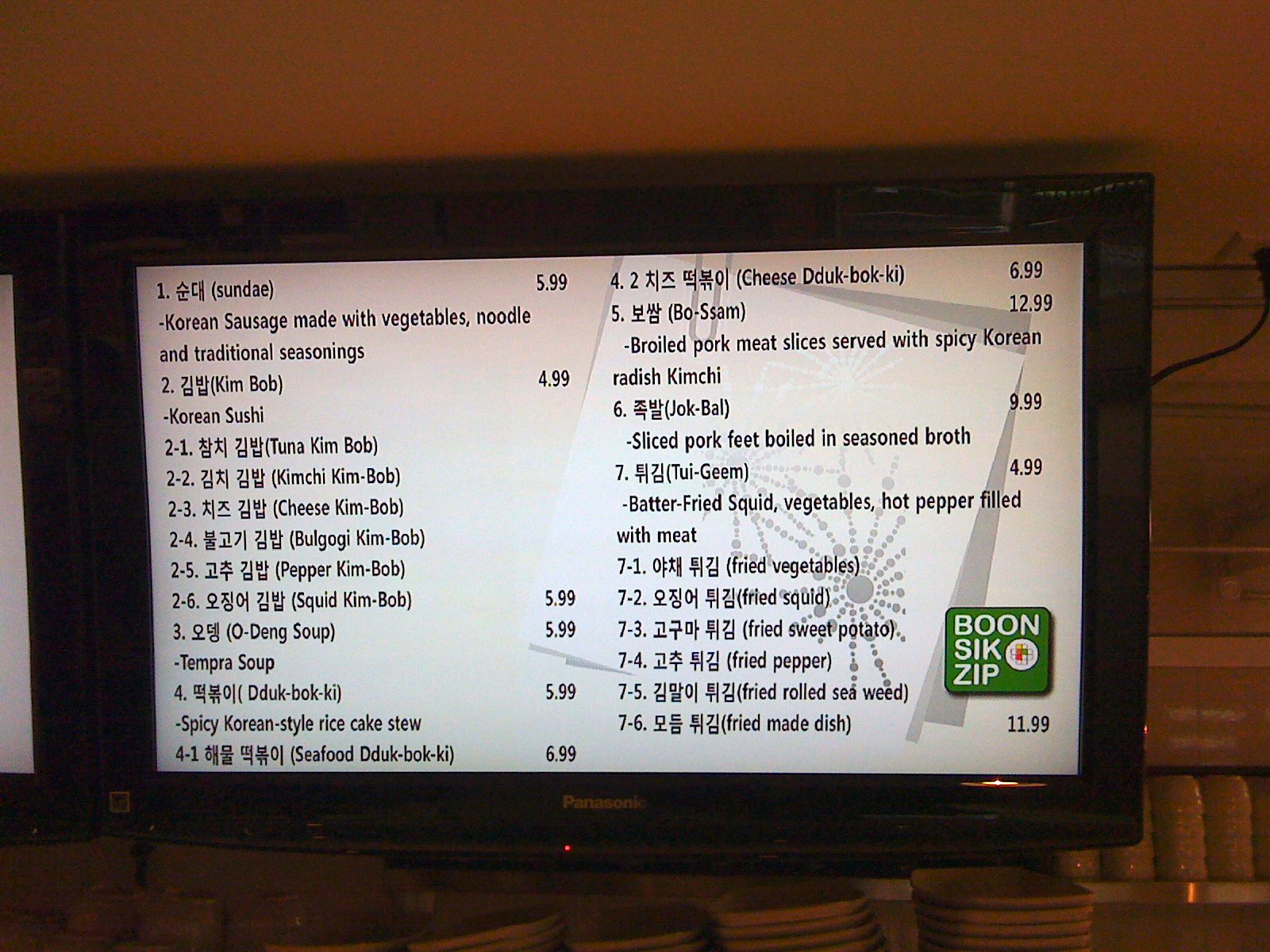This image features a digital menu displayed on a TV screen located inside a restaurant. The TV screen is prominently mounted against a wall that has a yellowish-red tint, covering the top inch of the background and descending down both the left and right sides of the frame. Just to the right side, at the bottom, the colored background extends underneath the TV. 

Behind the TV screen, a cord is visible, trailing slightly upward to the right, appearing to be plugged into the ceiling. Beneath the TV, a variety of items are organized. Close to the bottom right of the screen, there are multiple stacks of bowls: two full stacks are visible with a few more partially hidden under the TV. Above these bowls sits a red square with illegible text. 

In front of the TV, starting from the left side, there are three cups positioned on the counter. To the left of the power button on the TV, there is a small cluster of saucers: two stacked saucers, two more beside them, another set of four saucers, and finally, another four saucers—all of which are white. 

The TV screen itself has a black border. On the left edge of the image, the border of another TV screen is faintly visible. On the left side of the displayed screen, there is a list of sequential numbers: 1 2, 2 1, 2 2, 2 3, 2-4, 2-5, 2-6, 3, 4, and 4 1. Each number is aligned with a list of food items on the right side of the screen. Nearby, just left of the center, are various food prices listed in a sequence: 4.25, 6.7, and then from 7.1 down to 7.6.

Above the lowest price, a brown square contains a smaller green square with white lettering that reads "boon," followed by "SIK," and underneath that, "ZIP."